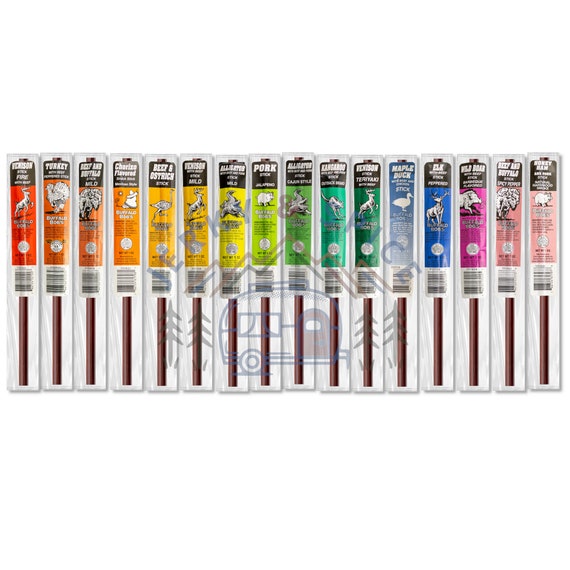This promotional image showcases an extensive product line of jerky sticks against a plain white background, designed to keep the focus on the products. The image features approximately 15 different jerky packages, each in varying vibrant colors that create a rainbow-like effect from left to right. The packages start in red and progress through multiple shades of orange, yellow, green, teal, blue, purple, and pink. Each package displays an animal graphic, suggesting the source of the jerky such as deer, turkey, buffalo, pork, elk, and duck, with specific color associations—red indicating deer, orange highlighting turkey and buffalo, yellowish orange, lime green for pork, and shades of green to blue and finally pink for various assortments like elk and duck. The design of each jerky stick includes a colored portion with animal imagery, a black label with white text, and a barcode below. A subtle watermark featuring a trailer logo and faint images of a camper and trees in the background hint at an outdoorsy, camping theme. The image likely aims to present the diverse product range to vendors or company stakeholders.